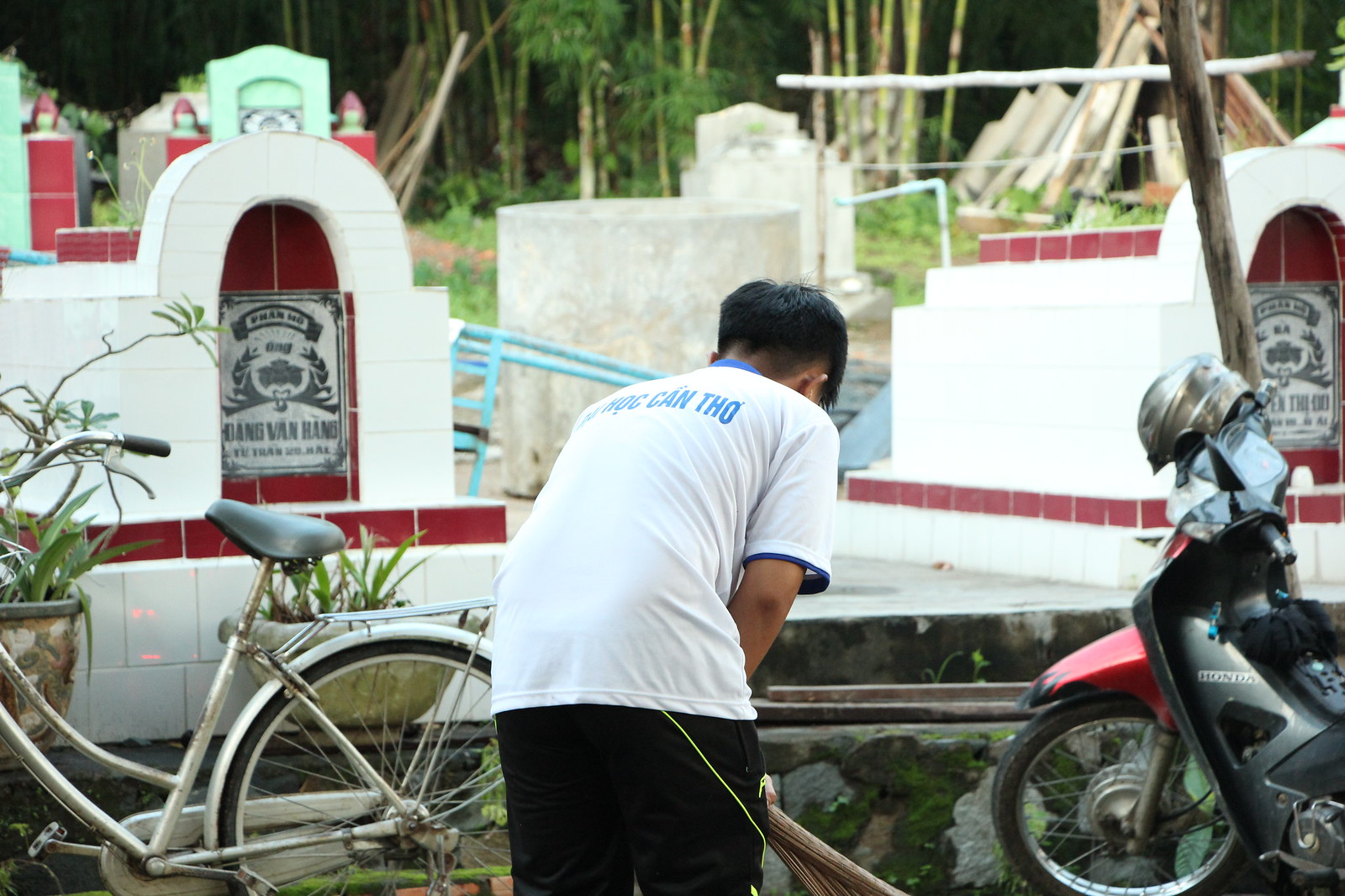In this rectangular image, a boy with light brown skin and black hair is seen from behind, intently fixing a light blue and gray bicycle positioned to his left. He is wearing a white shirt with blue collar and sleeve borders, adorned with partially visible blue lettering that reads "C-A-N T-H-O," and black pants with a neon green stripe. His torso is tilted to the right as he bends over, with his right elbow directed towards the bicycle's handle. To his immediate right, there is a red and black motorcycle topped with a silver helmet. In the background, multiple white and red glossy brick structures with smooth surfaces and arches are visible, reminiscent of gravestones or cemetery structures. Beyond these, there are hints of green vegetation, possibly bamboo trees or a forested area, as well as a makeshift teepee hut seen in the distance towards the upper right of the image.